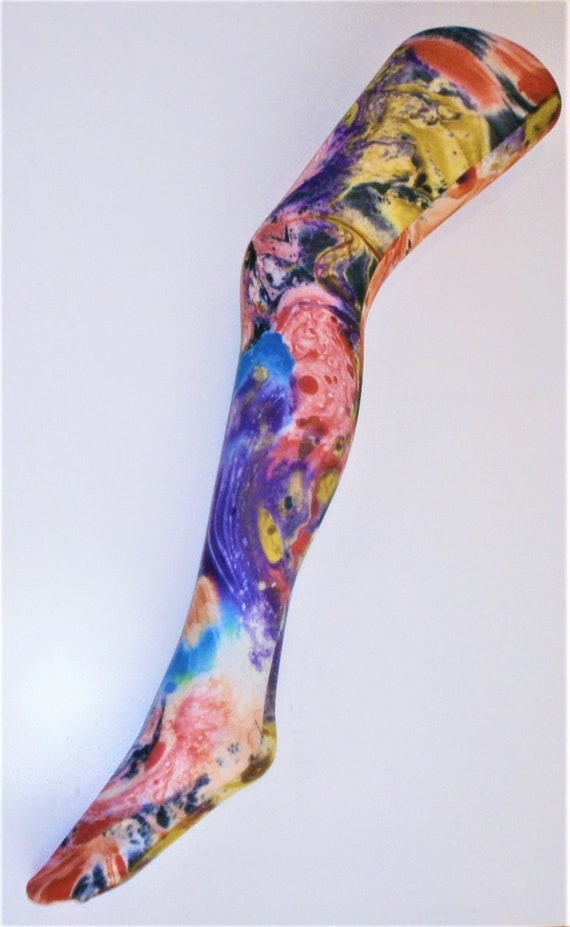The image features a close-up photograph of a mannequin's left leg adorned with a vividly colored, tattoo-like sleeve. The leg stretches diagonally from the bottom left corner to the upper right corner of a gray rectangular background. The sleeve, akin to a pantyhose, showcases a captivating cosmic design with a diverse palette of colors. Starting at the toes with shades of red, the pattern transitions into various hues of purple, blue, and accents of white, before evolving into darker tones of purples, blues, reds, and burgundies near the knee. Further up, the design incorporates earth tones such as yellow, green, light brown, and dark orange, creating an abstract, swirling motif reminiscent of a bowling ball pattern. The leg is slightly bent at the knee, enhancing the dynamic feel of the composition. The colors, though vibrant, have a slightly muted and aged appearance, blending together seamlessly and casting a faint shadow against the backdrop, adding depth to the image.